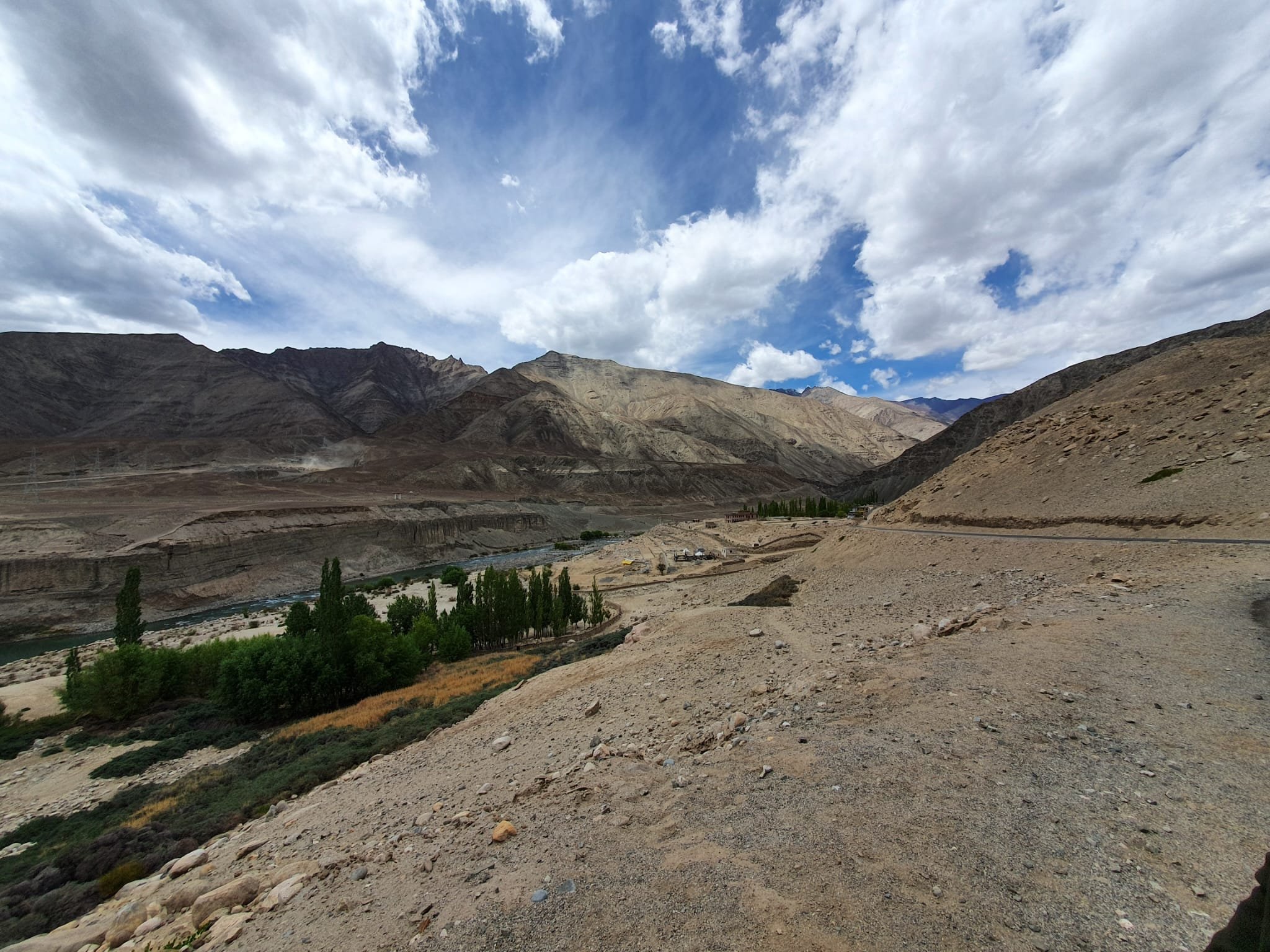The image is a colored photograph of a desert landscape featuring a strikingly blue sky filled with fluffy, white clouds. Below this expanse, a vast range of desert mountains stretches from left to right, displaying an array of earthy tones, including light browns, tans, and darker browns. The mountains' surfaces appear rugged and jagged, with noticeable differences in elevation, particularly on the right side. At the foothills of these mountains, a valley contains a river flanked by a small area of dark and light green trees, predominantly evergreens mixed with other shrubberies. The foreground transitions further into the dry, rocky desert terrain, littered with pebbles and larger stones, and the ground takes on a cream-colored hue amidst the scattered rocks and sand.